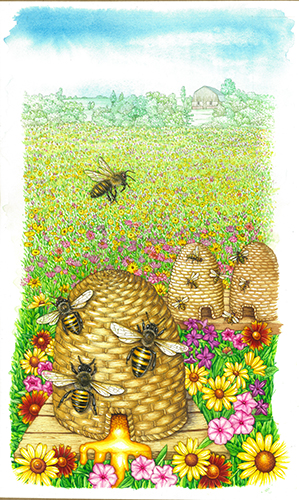The painting depicts a vibrant rural scene on a white background that fades softly at the edges. A lush green field, adorned with yellow, pink, and orange flowers, extends into the distance. In the right center of the frame, a rustic brown barn with a black roof stands against a pale green wood. Above, the sky transitions from white at the horizon to a medium blue at the top, dotted with clouds.

In the foreground, three stylized beehives, woven with a textured, golden beige material, are prominently featured. The largest hive on the left has three realistically painted bees with white wings perched on it, and another bee is seen flying above, wings raised and legs extended. A golden stream of honey trickles from the hive’s entrance. To the back right, two smaller beige hives teem with bees busily at work.

Overall, the scene intricately blends the tranquility of a flower-filled field, the industrious nature of bees, and the rustic charm of a countryside farm. The detailed flowers, including sunflowers, daisies, possibly pansies in varied hues of purple, yellow, pink, and red, highlight the pastoral beauty captured in the artwork.